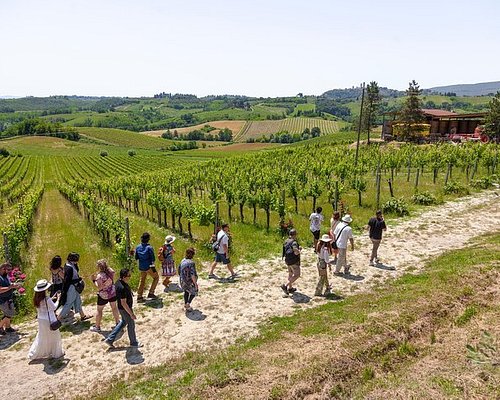This somewhat blurry photo, taken from above, captures a beautifully scenic vineyard in the countryside, which could be located in Australia, Italy, or Spain. The landscape extends far into the distance, showcasing vast fields of organized crops, potentially blueberry bushes, arranged in neat rows. The sunlit day highlights the rich greenery contrasted with the white pathway and earth underneath.

In the foreground, a diverse group of around ten tourists wanders along a white dirt trail that winds through the vineyard. These visitors, casually dressed and equipped with cameras and bags, comprise men, women, and children, some sporting sun hats. The path leads them up a slight hill, illustrating the vineyard's gentle terrain.

To the right in the distance stands a vineyard house, accompanied by a red building, likely a barn or shed, and a tractor that hints at the farm's functionality. This inviting scene is framed by meticulously plowed lands with sections of trees and patches of earth, extending across what appears to be hundreds of acres of largely flat, but slightly hilly, countryside.